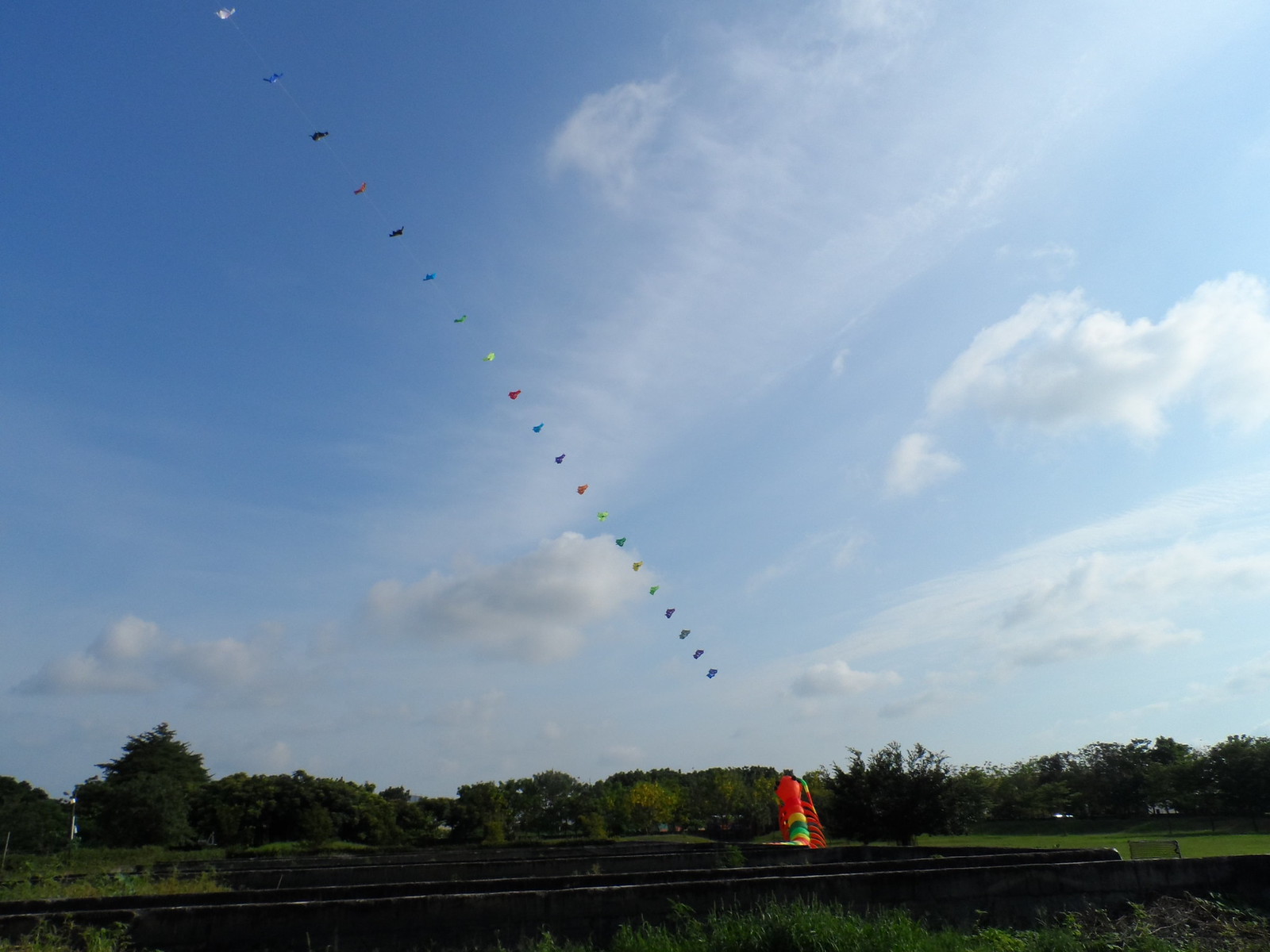The image showcases a vast, rural landscape under a blue sky filled with varying clouds, from fluffy white to those with a subtle gray undertone. Dominating the sky, a sequence of vibrant flags is strung along a line, displaying a spectrum of colors including white, blue, red, orange, green, yellow, and darker shades of red. This line stretches from an intriguing, multicolored object on the ground, which resembles a rainbow-colored or gummy worm-like figure, anchoring the flags. The ground features a mix of green lawn and scattered wooden pieces, possibly raised beds, as well as some dense tree lines in the distance. The foreground reveals what appears to be train tracks running through, hinting at an intersection between natural and man-made elements. A sign is posted on the lawn near the tracks, completing this outdoor scene.